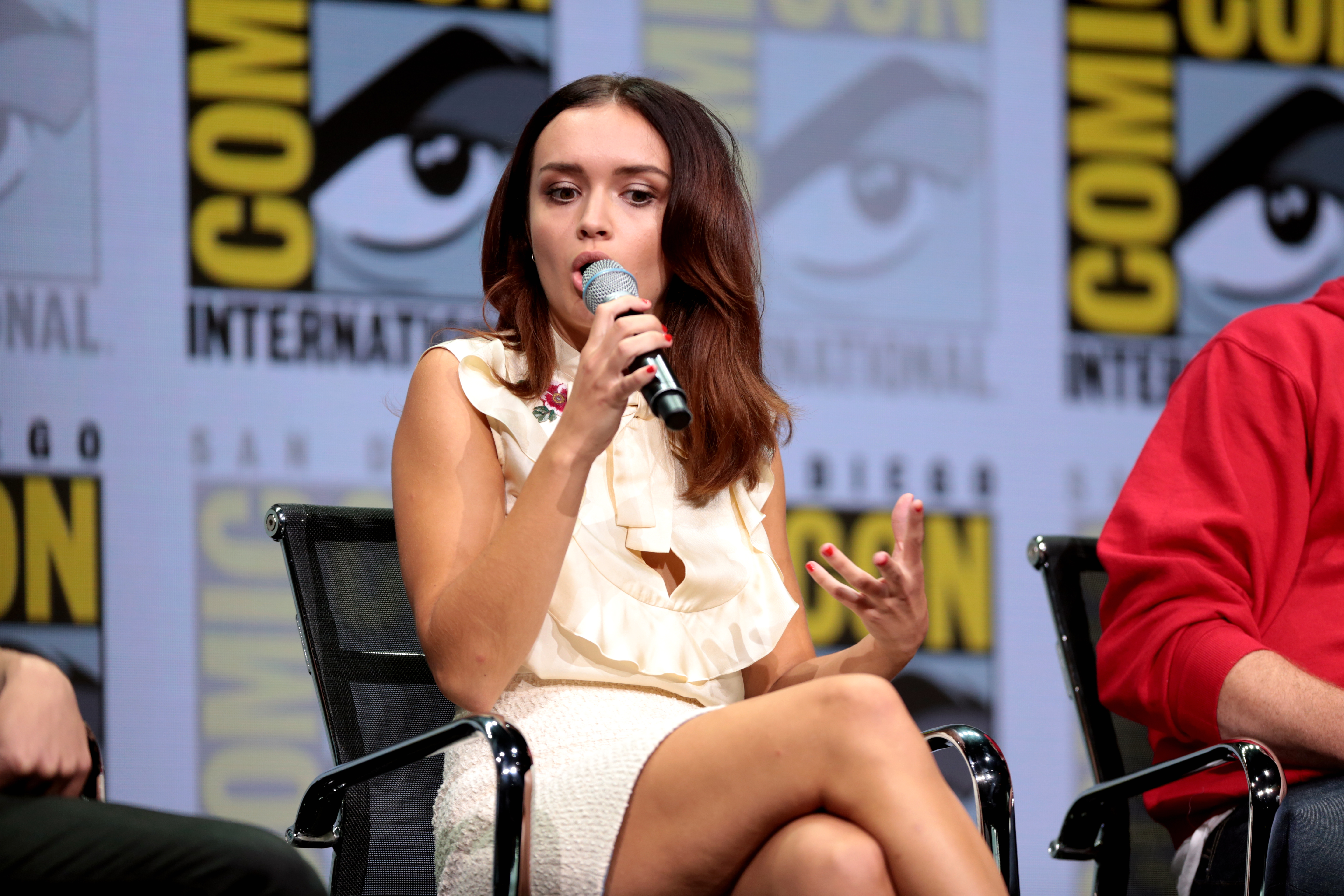The photograph captures a Comic Con event featuring a primary focus on a woman sitting center stage in a black mesh-backed metal chair. She is dressed in a short, denim-textured skirt and a sleeveless tan frilly top adorned with red and green floral patterns. The woman has dark brown hair and holds a microphone close to her face, partially obscuring it. The background includes a banner for Comic Con, though its exact color isn't clear. To her right, there is a person partially visible, identifiable only by the side of their body, wearing a long-sleeved red shirt with rolled-up sleeves and blue jeans. On her left, part of another individual’s leg and hand can be seen, dressed in black pants. The setting is somewhat dim, emphasizing the detailed attire and seating arrangements of those visible in the image.